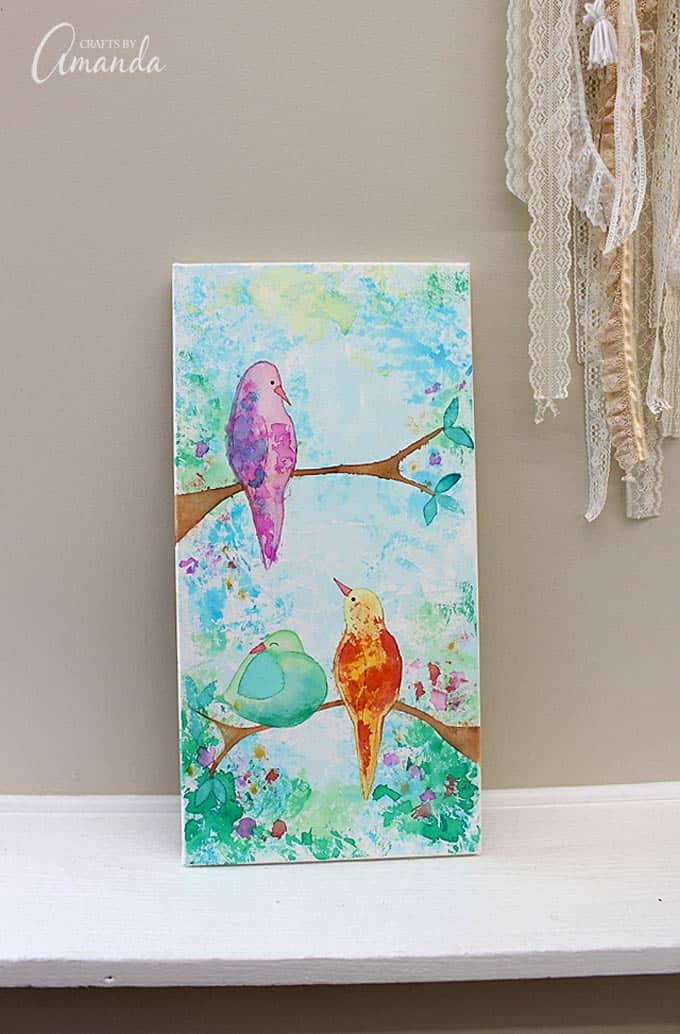The image features a vibrant, watercolor painting of birds perched on tree branches, displayed against a tan wall on a white shelf. The notecard-sized painting is oriented vertically, with its shorter side at the base. In the top left corner, white lettering spells out “Crafts by Amanda,” while the top right corner showcases cream, white, and tan lace ribbons hanging down.

The painting itself depicts an intricately detailed scene with two tree branches. The upper branch, entering from the left side and adorned with green leaves at its tip, hosts a pink and purple bird with an orange beak, facing right. The lower branch, extending from the right side, features two birds: one orange and yellow with a pinkish beak, and the other green and blue, both facing left. One of the birds appears to be washing itself.

The background of the painting is a beautiful melange of vibrant colors, including splattered shades of blue, green, and a touch of purple. The entire image is brightly lit, providing clear visibility and highlighting the detailed artistry of the scene.